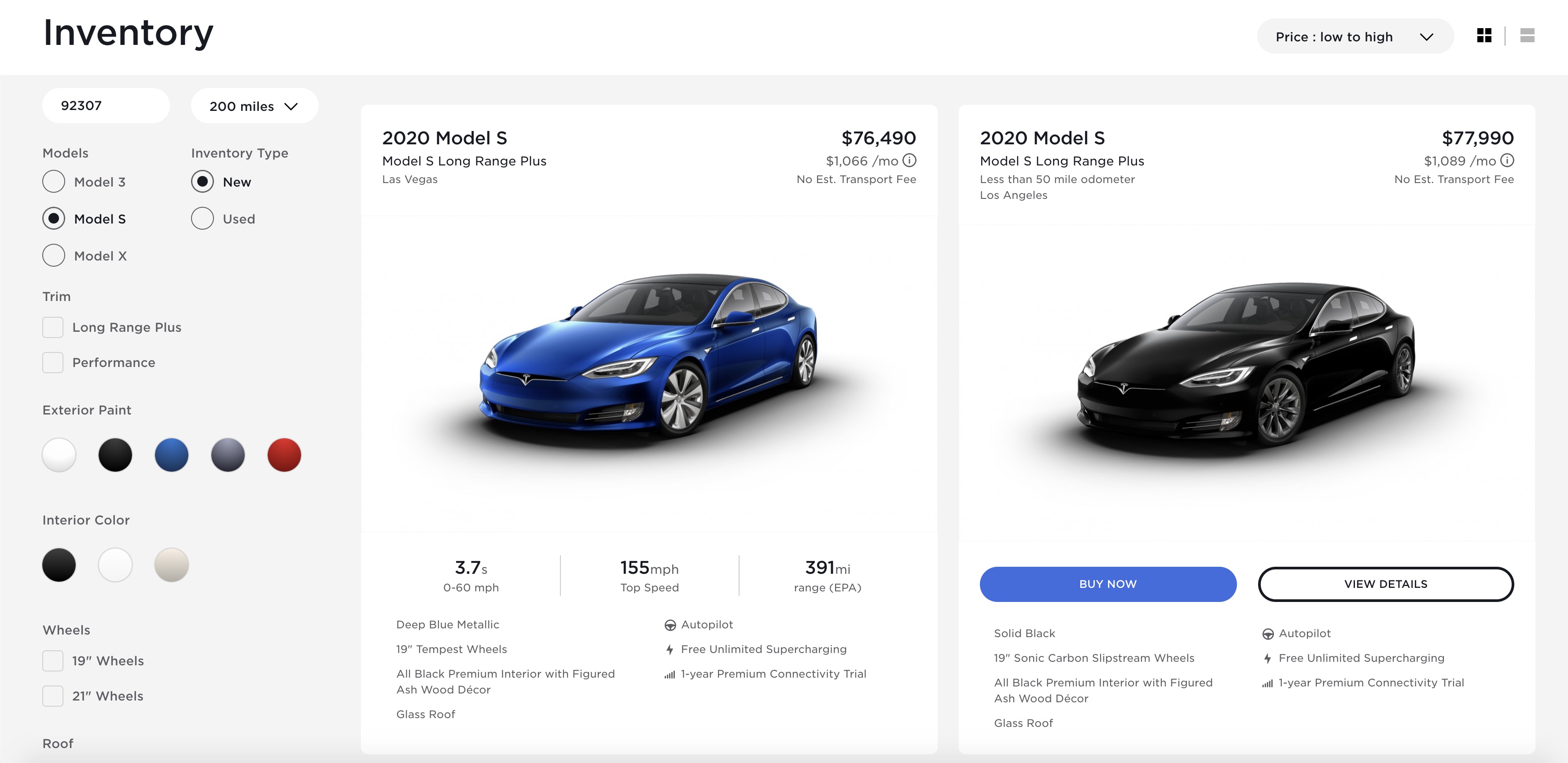This image is a screenshot from a car website's inventory page. At the top left, "Inventory" is displayed in black font. To the right, there's a drop-down menu labeled "Price: Low to High." 

The main section of the webpage is divided into two columns. On the left side, there are several filtering options. At the top, there's an entry code "292307" and a selected range of "200 miles." Below this, the available filters include:

1. **Models**: Options include Model 3, Model 5, and Model X.
2. **Inventory Type**: Choices between New and Used vehicles.
3. **Trim**: Options for Long Range Plus and Performance.
4. **Exterior Paint**: Available colors are White, Black, Blue, Grey, and Red.
5. **Interior Color**: Options are Black, White, and Beige.
6. **Wheel Size**: Choices between 19-inch and 21-inch wheels.
7. **Roof Options**: The remainder of this section is cut off in the image.

On the right side, there are two car listings. The first car is a 2020 Blue Long-Range Plus model priced at $76,490. The second car is a 2020 Black Long-Range Plus model with a price tag of $77,990.